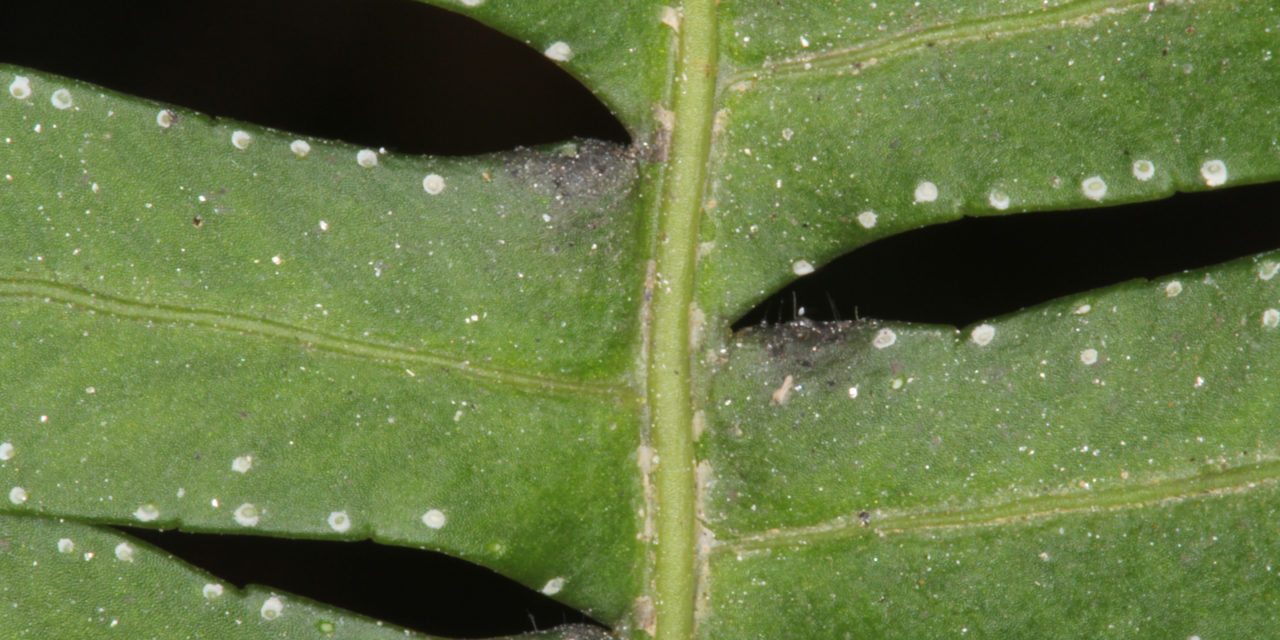This rectangular and highly detailed photograph presents a close-up, likely microscopic, view of a leaf. The image centers on the leaf's prominent, lighter green spine or main vein, from which smaller veins branch out symmetrically to the left and right. The leaf exhibits a range of green shades, with the main vein being lighter and the surrounding foliage darker. A distinct feature of the leaf is the presence of several large, teardrop-shaped holes, two on the left and one on the right. These holes, possibly the result of insect damage, are surrounded by numerous small, white dots spaced intermittently and somewhat regularly along their edges, which may indicate a type of growth or reaction to the damage. Additionally, the picture displays various shadows and shading, including almost black, fish or whale-shaped shadows and some tan areas that might be due to dirt or other natural elements. The intricate details and varying textures, including what appear to be tiny hairs or cilia at the intersections of veins and holes, underscore the complexity and beauty of the plant structure captured in this image.